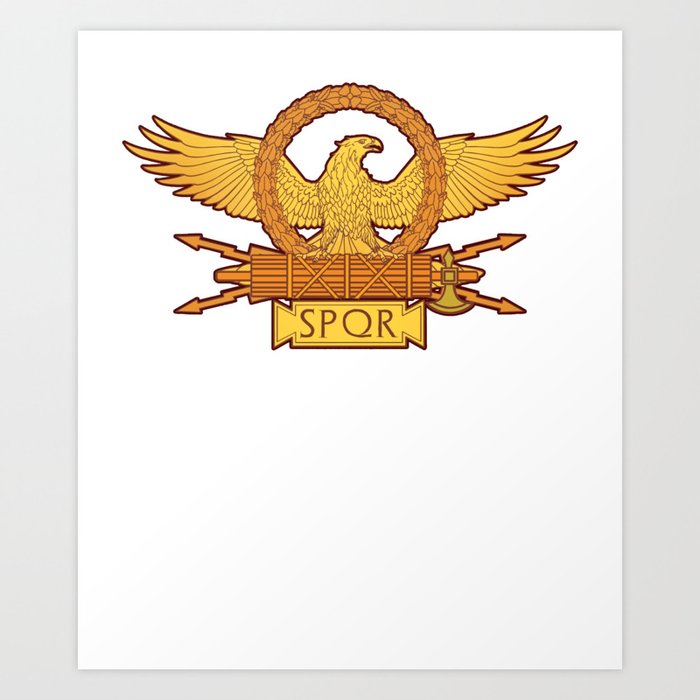The image presents a vertically rectangular artwork bordered by a thick gray frame on the sides and thinner on the top and bottom, with a white interior background resembling a piece of paper. Centered in the upper half is a vibrant logo primarily in shades of yellow and orange. The focal point is a majestic yellow eagle with outstretched wings displaying pointed, sharp feathers. The eagle faces the right and stands firmly on a horizontal orange pole. At each end of the pole are arrow-like extensions pointing outward. The eagle's talons grasp this pole, around which weapons, possibly including arrows and lightning bolts, are bundled. Surrounding the eagle, a bronze wreath encapsulates its torso, though its expansive wings extend beyond this circular frame. Below this compelling image, inscribed in yellow, is the term "SPQR," standing prominently at the base of the composition. The contrasting background of the white canvas against a grayish wall highlights the logo's rich, warm hues of yellow, orange, and the darker tones of brown.